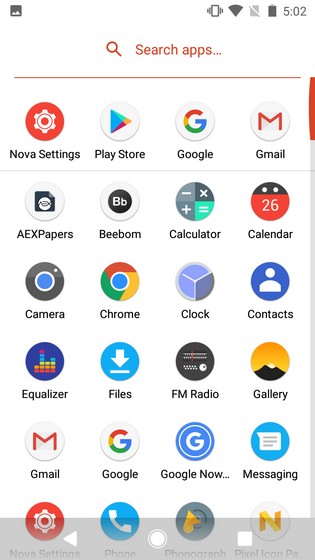The image is a screenshot from a smartphone displaying an apps page with a white background. The upper right corner shows the time as 5:02, though it doesn't specify AM or PM. The battery icon appears fully charged, alongside the Wi-Fi icon and a mute icon. 

At the top center, in red font, the screen reads "Search apps" with a search icon—a circle with a diagonal line—on the left. Beneath this text is a red line separating the search bar from the rest of the screen. 

The app icons are arranged in a grid, four across and six down. The first row includes:
1. **Nova Settings** - represented by a red circle.
2. **Play Store** - depicted as a pyramid shape with the signature Google colors.
3. **Google** - symbolized by a "G" in Google colors (red, yellow, green, blue).
4. **Gmail** - illustrated by an older icon with a red "M."

Subsequent rows contain a variety of app icons, each distinct in color and design:
- **Camera app** - a blue circle with a black border.
- **Clock app** - designed like a pie chart, two-thirds light blue and one-third gray.

At the bottom of the page, the border is a very light gray, overlapping the icons in the last row, which includes:
- **Phone app** - identifiable by its traditional icon.
- **Another app** identifiable only by a gold-colored "N."